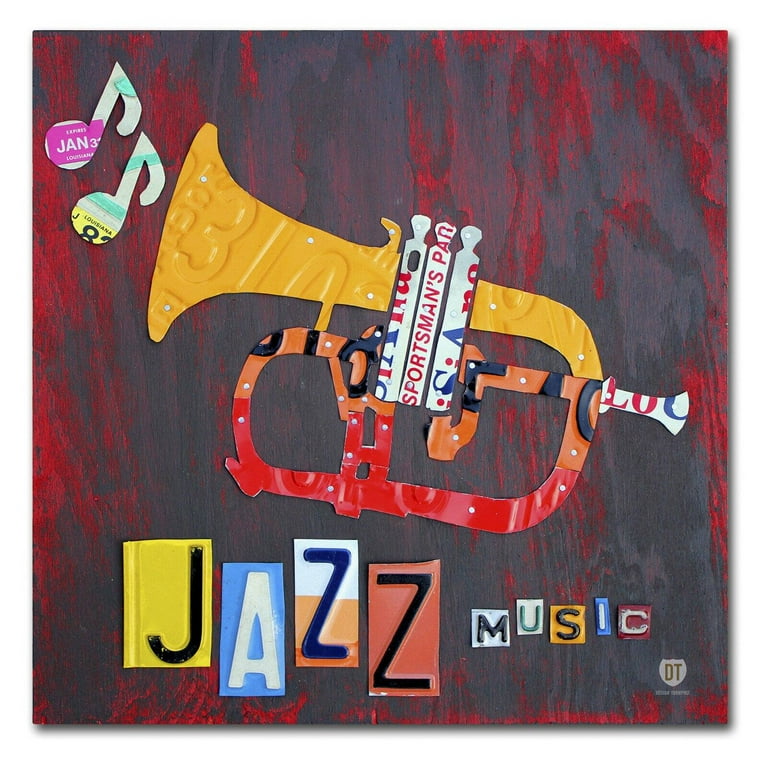This piece of artwork marries rustic charm with a musical tribute through a unique medium — license plates. Set against a vividly stained and distressed wooden background dominated by shades of red and black, the collage features meticulously crafted elements. To the left, two white musical notes with green striping, likely from the same plate, bear the inscriptions "January 31st" and part of an '8'. Dominating the center, a trumpet-like instrument, composed of fragments of various license plates, showcases intricate details: a yellow horn cone juxtaposed with different colored sections for the remaining parts. Notably, the three pads for the buttons and the mouthpiece are distinctly visible. The words "jazz" and "music" are prominently displayed using an eclectic mix of larger and smaller letters cut from assorted plates, evoking a patchwork aesthetic akin to a ransom note. Each letter's color varies, flaunting hues of yellow, blue, white, orange, reddish-orange, and whitish-green, adding vibrancy to the piece. At the bottom, a shield bearing the initials "DT" — presumably the artist's signature — anchors the artwork, which is tacked down with small, flat-headed metal pins, solidifying its handcrafted appeal.